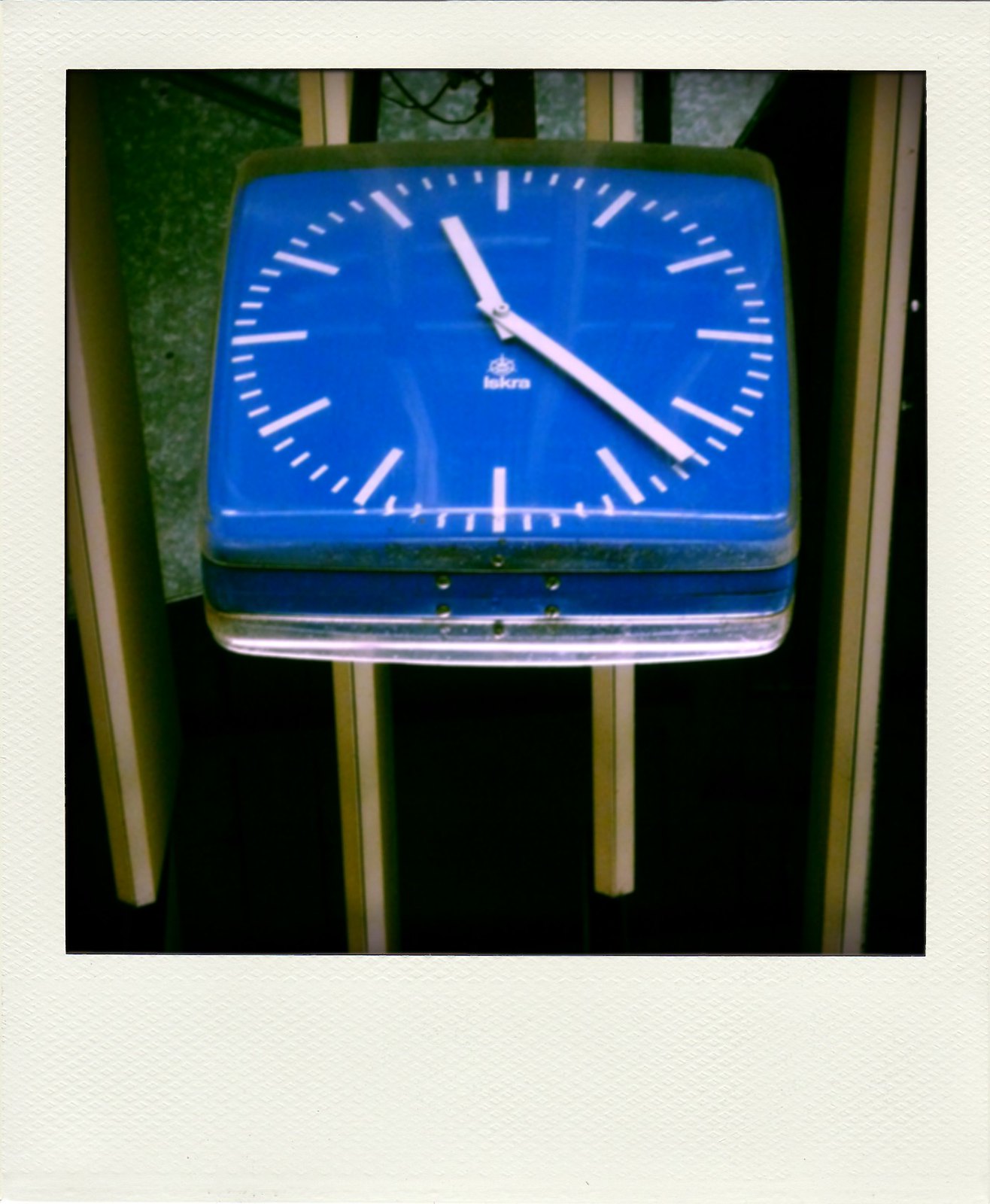This photograph captures a distinctive analog clock with a clear blue face marked by large white lines for the hours and smaller white lines for the minutes, notably without any numerical markings. At the center of the clock, below the white hands displaying the time as approximately 11:22, is a logo and the brand name "ISKRA" prominently displayed. The clock appears quite large and has a rounded and slightly scuffed edge, indicating wear. It also features a multi-layered external body and is encased in plastic. The clock is either mounted or positioned in an ambiguous manner, as it seems to be hovering within the image. The background is a mix of lighter sections at the top, with metal visible, and darker tones below, divided by a set of vertical wooden beams or panels. The photograph itself is framed by a cream-colored border, grounding this visually intriguing depiction of the clock within its context.